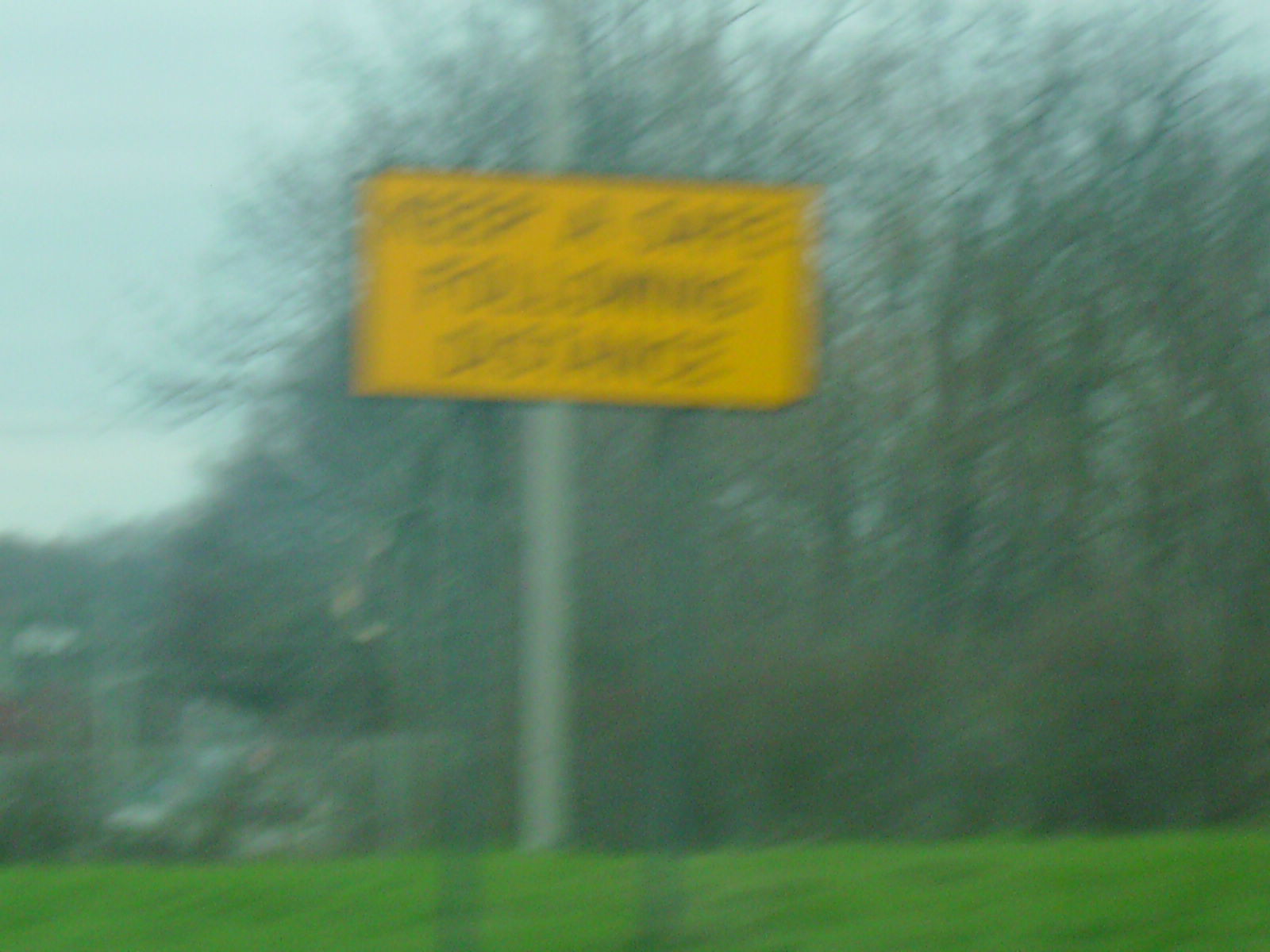This outdoor photograph captures a scene dominated by a pervasive blur, likely caused by camera movement. In the background, a partly cloudy blue sky stretches above a distant mountain or hilly range, which is visible on the left side of the image. The mid-ground is filled with a tree line, primarily brown and devoid of leaves, revealing bare branches and trunks grouped together. The bottom strip of the image features a vibrant green grassy area extending across the frame. Centrally located in this grassy area, a gray metal pole supports a prominent, bright yellow rectangular sign that reads "Keep a Safe Following Distance" in black print, though the blur makes the text hard to discern. The overall composition suggests a roadside setting, with the sign serving as a safety reminder amidst the natural, albeit blurred, scenery.